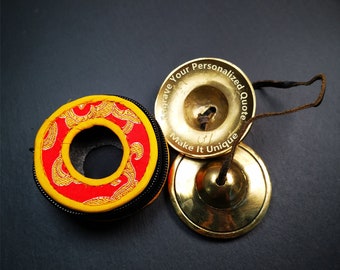The image features three objects arranged against a dark gray, almost black background. To the left, there is a round, zippered storage case adorned with intricate Asian-inspired designs. The case is predominantly red with yellow accents, including a yellow fringe around its exterior and another inner yellow band, creating a striking visual contrast. Among this red section with yellow markings, notable patterns appear: one spans the top edge from left to right, another is situated in the upper left corner, a third is on the lower left, and a final significant design is on the bottom right.

To the right of the case are two brass finger cymbals, small and circular, linked together by a brown leather cord threaded through their centers. One cymbal is face-up, displaying the phrase "your personalized quote, make it unique" in white, seemingly engraved along its rim. The other cymbal is face-down, partially tucked under the first, with a raised center where the connecting string is visible. These cymbals are instruments typically held in the hand and clashed together to produce sound. The composition and design elements reflect a blend of functionality and aesthetic appeal, likely serving both practical and decorative purposes.